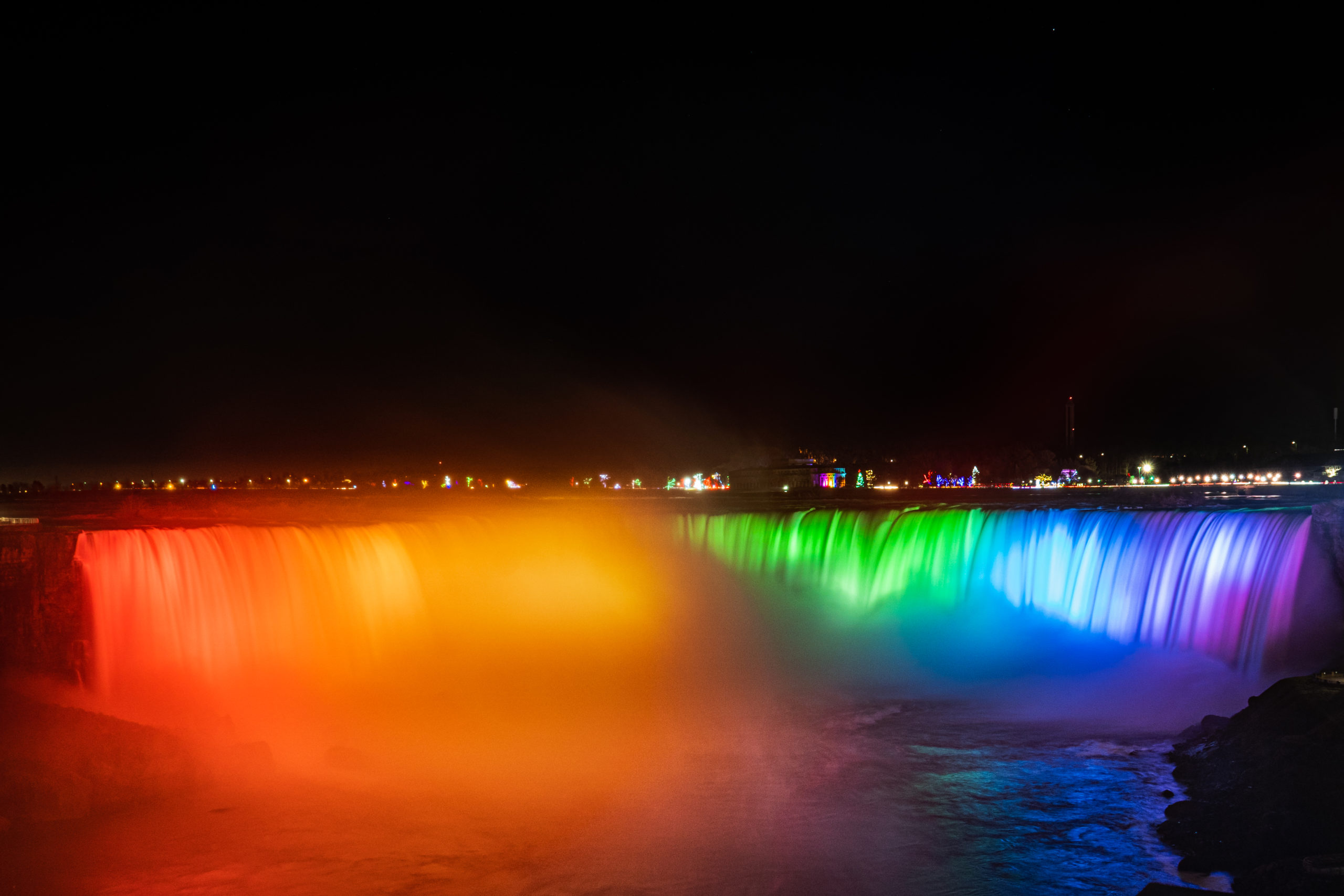This rectangular photograph captures a breathtaking nighttime scene outdoors. Dominating the foreground is a grand, cascading waterfall, likely Niagara Falls, illuminated with a spectacular array of fluorescent colors. From left to right, the waterfall transitions seamlessly through red, orange, green, blue, and purple hues. The vibrant illumination highlights the waterfall's powerful descent, with a thick mist and foggy spray rising where the water crashes into the lower basin. The backdrop features a pitch-black sky devoid of stars, setting a stark contrast to the lively cityscape on the far side of a large body of water. The city's lights twinkle and dance along the horizon, adding an additional layer of brightness and color to this mesmerizing nocturnal vista.